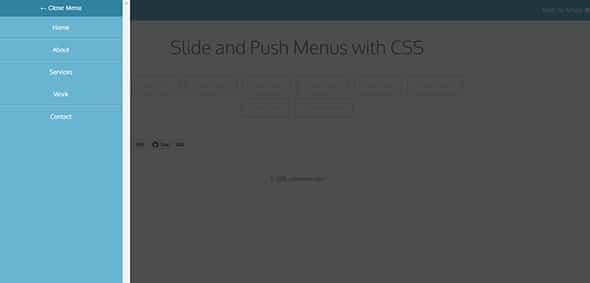The image features a light blue background with a variety of textual elements. In the top left corner, the slightly blurry text "CheapMama" is accompanied by an arrow pointing to the left. Beneath it, vertically aligned white text reads: "Home," "Cool," "Services," "Wire," and "Contact," each separated by horizontal lines.

Dominating the center-right of the image, a darker tinted area features the words "Slide and Push Menus with CSS." Below this heading, there are eight small rectangular boxes, arranged with six on the top row and two on the bottom row. Additionally, on the bottom left, there is some black text which is not clearly legible.

A long horizontal blue bar runs across the top of the image, with some white text in the top right corner. The bottom sections of the image — middle, left, and right — appear to have empty spaces. A scrollbar is visible along the middle left side of the image, indicating that there might be more content not currently in the visible area of the image.